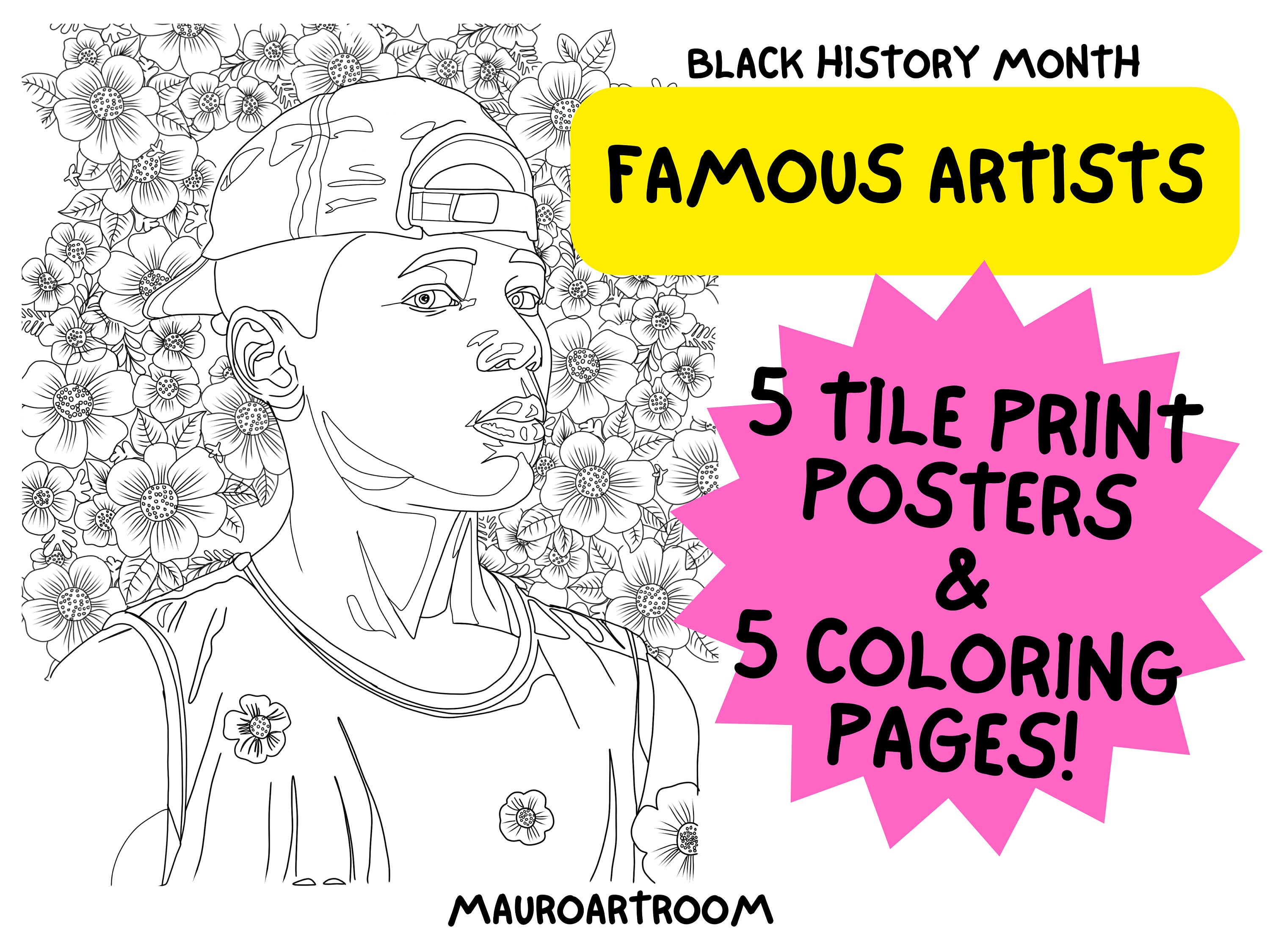This detailed flyer or poster, designed to celebrate Black History Month, features a black and white pen-drawn illustration of a young African-American man. The man is depicted wearing a backwards baseball cap and a sleeveless tank top adorned with floral sketches. In the background, an intricate array of flowers also drawn in pen highlights the artistic design. Positioned on the right side of the poster, the words "Black History Month" are prominently displayed above a yellow rectangle containing the text "Famous Artists." Beside it, a pink starburst catches the eye with the announcement "Five Tile Print Posters and Five Coloring Pages!" At the bottom center of the poster, the text reads "Morrow Art Room," indicating the source or sponsor of this artistic celebration. Inspired by the style of Kehinde Wiley, this flyer serves as a vibrant example of racial and cultural appreciation through art.